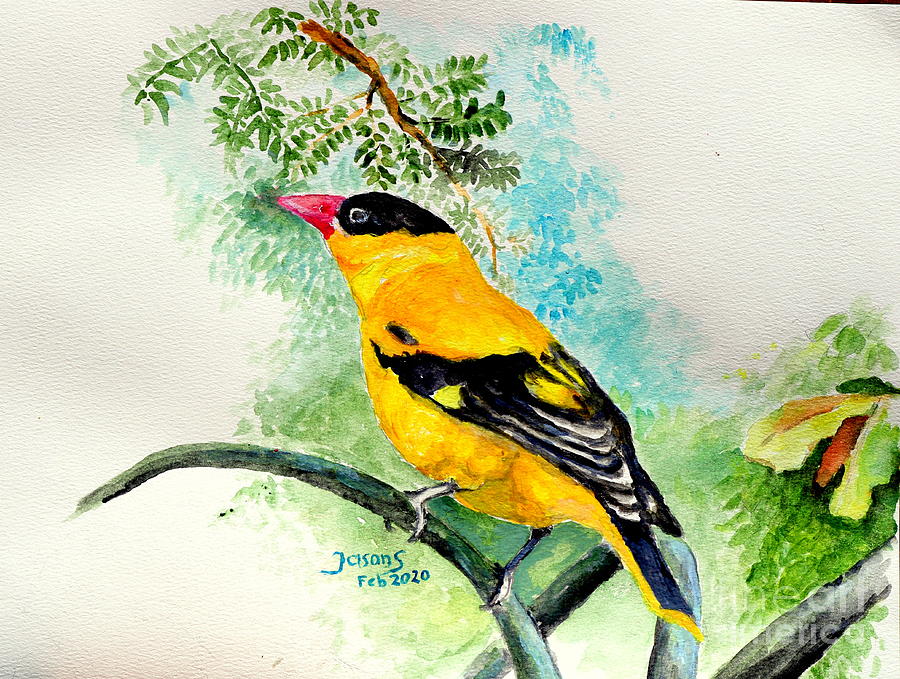The image showcases a detailed watercolor painting on a cream-colored canvas, signed "JASANS, February 2020" in blue at the bottom. It features a vibrant yellow finch with a distinctive black crown and black-tipped wings and tail, adorned with white and gold markings. Its red, comb-shaped beak adds a striking contrast to its brightly hued body. The bird, perched on a gracefully curved branch, faces west, clutching the branch with its small legs. Surrounding the bird are various watercolor elements: blue-hued plants and foliage in the background, a second branch set back further above the bird's head, and a distant branch adorned with small green leaves. Additional green grass softly painted in the lower right corner adds depth to the scene. The painting includes a partially legible watermark in the bottom right corner, possibly reading "Time Art America."